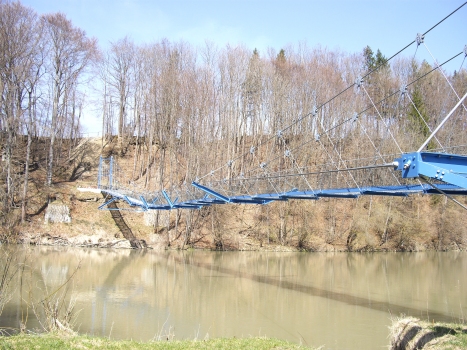The image captures an outdoor, wilderness scene featuring a wire suspension bridge extending across a wide river. The perspective suggests the photo was taken from the shoreline below, emphasizing the bridge's suspension system with white or silver wires and ropes. The bridge, possibly intended for foot traffic due to its size, spans from the left side to the right, supported by the intricate web of steel bars and cables. The lower half of the image presents the calm river, bordered by patches of green grass. Central to the frame is a tall, rugged cliff of tannish-brown dirt with a densely wooded hill above it, showcasing rows of leafless trees, indicative of a fall setting. The sky above is a mix of light blue and white, completing the serene, natural vista with hues of blue, gray, white, brown, and green. There is no text present in the image.